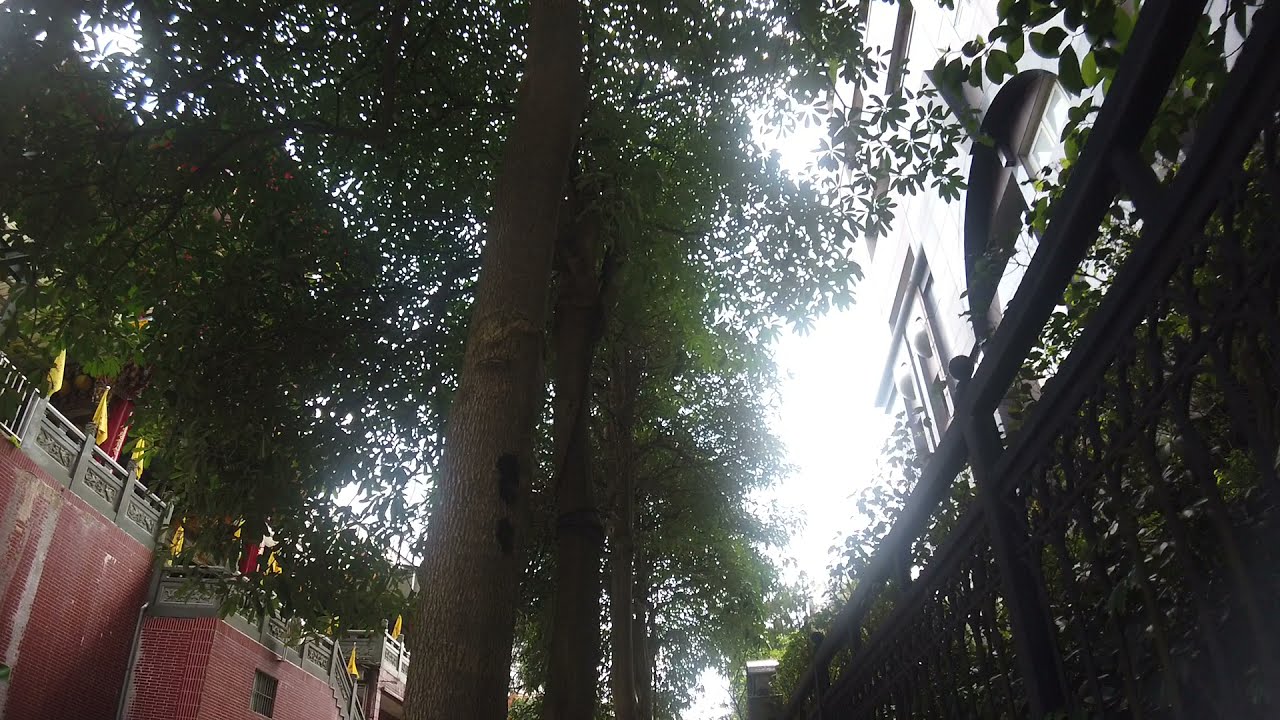This photograph, taken from the ground looking upwards, captures the majestic canopy of tall trees with thick, cylindrical trunks and abundant green deciduous leaves. The trees dominate the center of the image, creating a lush, expansive overstory. To the right side of the photograph, a black wrought iron fence runs parallel to the trees, partially obscured by green bushes. Beyond this fence, a sizeable gray stone building with an elegant facade is barely visible through the foliage, adding a touch of grandeur to the scene.

On the left side, a striking red brick wall ascends approximately 40 feet, topped by a gray fence, which seems to serve as a protective barrier. A stairway climbs up to this elevated walkway, suggesting that the wall might be part of a larger complex, possibly a castle or shrine. Decorative yellow and red flags line the top of the wall, adding a splash of vibrant color to the otherwise earthy tones. 

The photograph, wider than it is tall, emphasizes the towering height and expansive spread of the trees' canopy, creating a tranquil and almost reverent atmosphere under the leafy cover.